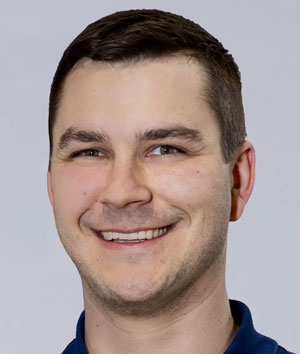This image is a vertically-oriented, rectangle-shaped photograph focused on a man who is smiling widely, displaying an open-mouthed grin that reveals his top row of teeth. The man, who is Caucasian, has short, close-cropped dark brown hair and a bit of stubble, giving him a five o'clock shadow look. His right eye is more squinted than his left, and both eyes seem to have a lighter color, possibly blue, gray, or greenish, although they're not particularly dark. He has relatively large eyebrows and a joyful expression that makes his eyes squint up. The photograph captures him from the neck up, showing just the top of his collar, which appears to belong to a collared navy blue shirt. The background is a solid gray, enhancing the focus on his happy facial expression.